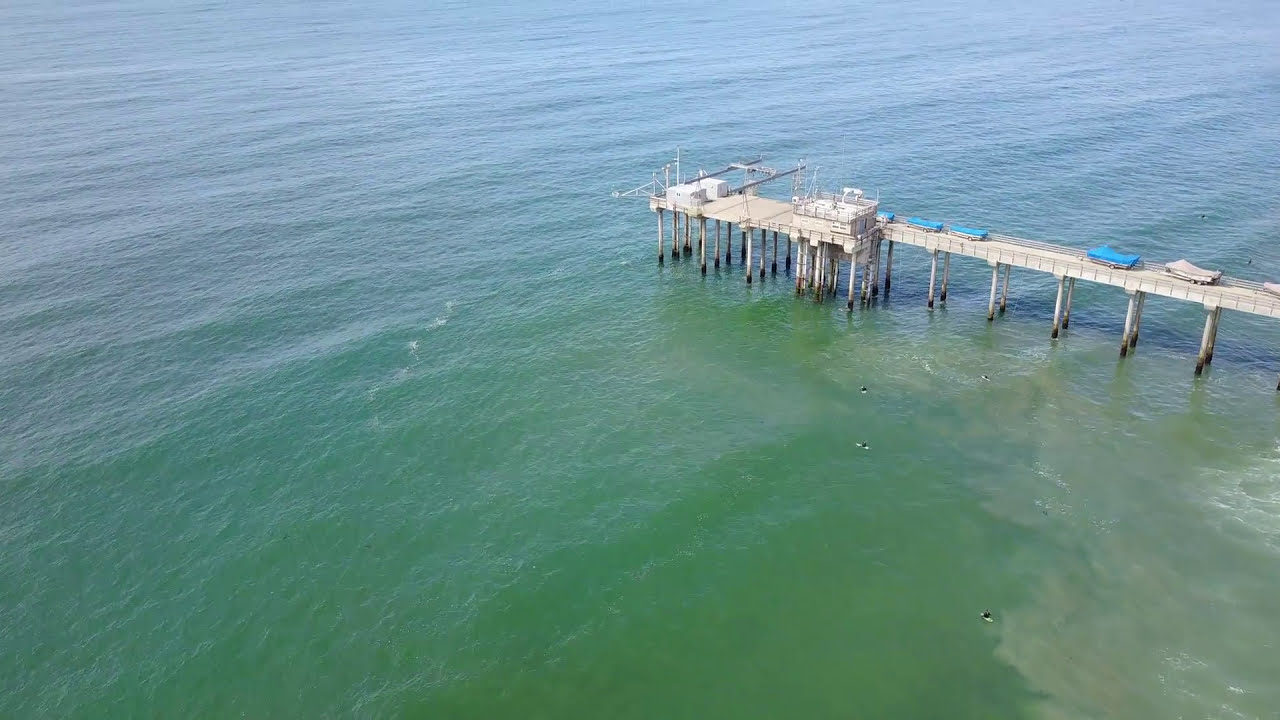An aerial shot captures a cement dock on the right-hand side of the image, extending at an angle toward the center. The dock is primarily gray and white and supported by multiple cement pillars. Various boats are lined up along the dock, covered with blue, gray, and teal tarps, and there appear to be two jet skis in the back with known shapes. A crane is stationed at the end for lowering items, and a small building equipped with fencing and utilities occupies the far end. The surrounding water transitions from medium blue in the upper right to a sea green hue towards the lower right, with noticeable patches of muddy water near the dock. The overall scene suggests a functional pier, possibly intended for shipping or business operations rather than leisurely activities.